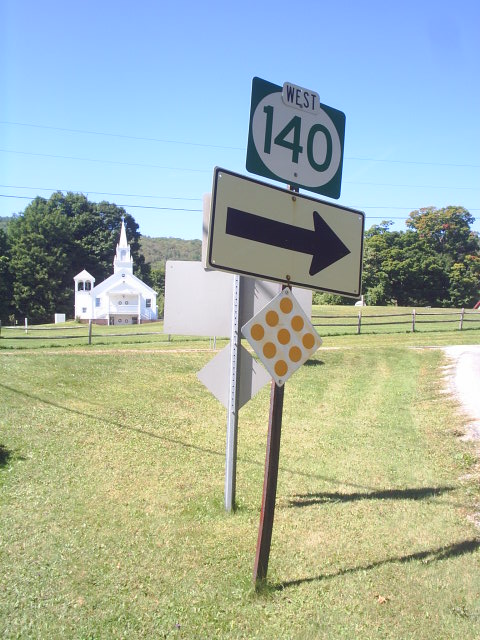This daytime photograph captures a scene dominated by a collection of road signs mounted on metal posts in the center. The forward-facing signs include a lower panel with a white background and orange dots, a middle panel featuring a white background with a black square and black arrow, and an upper panel displaying a darker color with the number 140 in a white circle. Above this, the word "West" is printed in black against a white background. The white backs of other signs are also visible. Surrounding the signs, a variety of shades of green, yellow, and brown short grass can be seen, along with a wooden fence. Behind the fence stands a white church building, and beyond that, a backdrop of trees in varying shades of dark and light green is visible. The upper part of the image shows power lines stretching across a clear blue sky, completing this intricate and detailed roadside tableau.